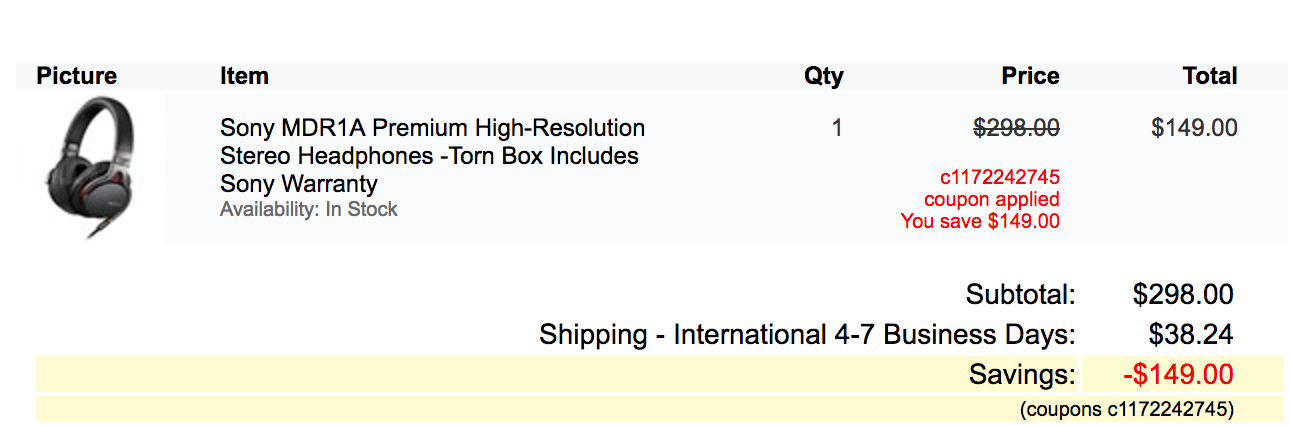The image displayed is a partial screenshot from an e-commerce website featuring a specific product listing. The background is white, providing a clean and uncluttered layout. The top of the section seen in the image is labeled "Item," aligned to the left.

The product listed is the "Sony MDR-IA Premium High Resolution Stereo Headphones." Details mention that the box is torn but includes a Sony warranty. An accompanying black and white image of the headphones is positioned to the left, showcasing the over-ear design in various shades of gray.

To the right of the image, the following information is provided:
- **Quantity:** 1
- **Price:** Originally $298, with a line striking through it to indicate a discount.
- **Coupon Applied:** In red font, showing a savings of $149.
- **Total:** $149
- **Subtotal:** $298
- **Shipping:** $38.24

A highlighted deduction of $149, once again in red font, is applied to the total cost.